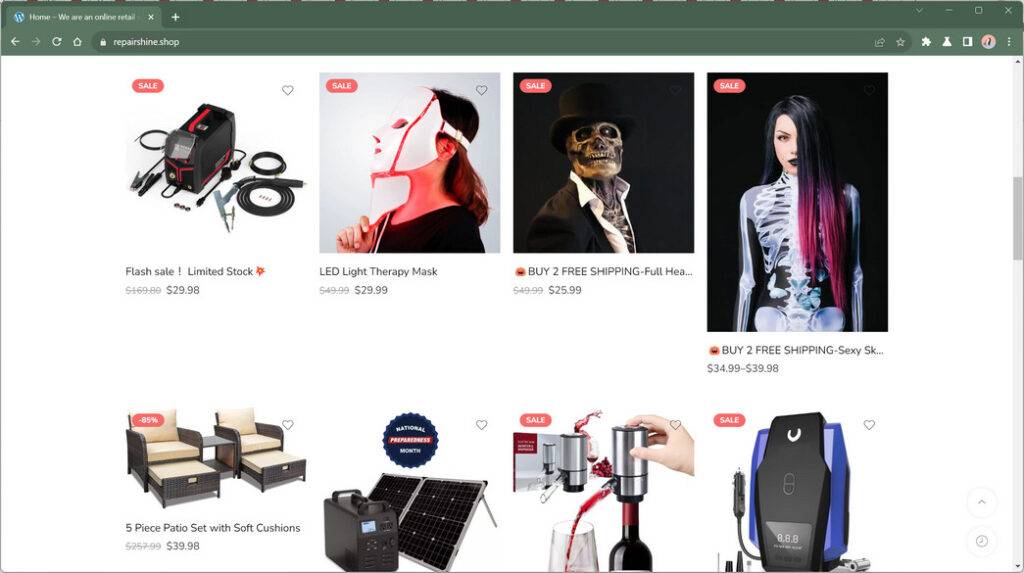**Detailed website screenshot description:**

The image is a screenshot of a webpage, specifically an e-commerce site, with the partial URL "repairshine.shop" visible. The screenshot captures the browser interface along with a section of the webpage. The browser's top bar is green, which indicates it is part of the user's computer theme, not the website itself. In the browser's top bar, various elements are visible, including browser tabs, the URL field, a few browser extensions, and navigation buttons such as the home, forward, and backward buttons.

Moving to the webpage content, the visible portion showcases a collection of items, arranged in a grid format. Although the webpage is partly cut off, it displays eight products in total, organized in two rows with four items each. In the first row, the following items are displayed from left to right:

1. **LED Light Therapy Mask:** The description mentions it being a "Flash Sale Limited Stock."
2. **Unidentified Item:** Appears to resemble a charger or battery, but the text is unclear.
3. **Halloween Masks:** A couple of masks suited for Halloween festivities are visible.
4. **Another Halloween-related Mask:** Similar to the other mask display, contributing to the Halloween theme.

In the second row, the following items are displayed from left to right:

1. **Five-Piece Patio Set with Soft Cushions:** This includes a photo showcasing two chaise lounges arranged attractively, denoting a comfortable outdoor furniture set.

The screenshot cuts off after these eight items, preventing us from seeing the entire page. The image thus provides a limited but detailed glimpse into the e-commerce site’s product offerings, emphasizing a mix of seasonal items and household products.